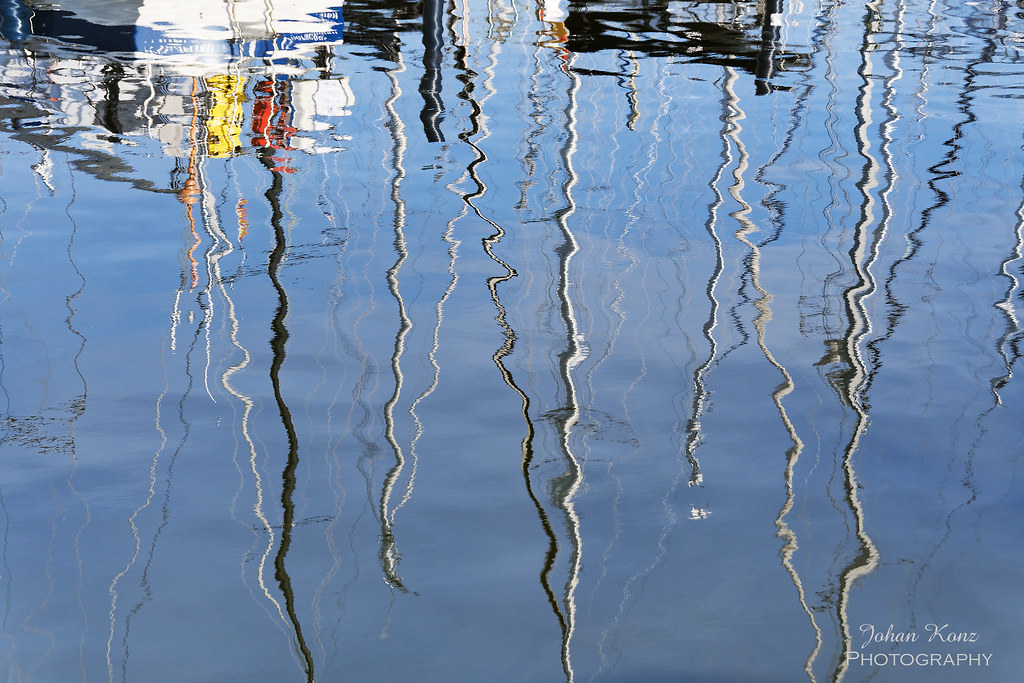This photograph, enclosed within a rectangular frame, captures the delicate interplay between water and light. The scene features still, slightly rippled blue water, reflecting a series of boats. The boats, which lie horizontally along the top edge of the image, have masts that extend downwards into the water, giving an inverted appearance. The masts are distorted by the water's subtle waves, creating crooked, wavy lines in white, black, and some outlined in both colors. These lines, though originally vertical, are broken and fragmented by the water's surface, resulting in an array of diagonals and zigzags. The boats themselves appear to be primarily white, with some featuring additional colors such as blue, red, yellow, and black. No sails are visible, only the ropes draping down from the masts. The impressionistic effect of the water's ripples makes the image resemble a pastel drawing. In the lower right corner, the watermark "Johan Kanz Photography" is elegantly inscribed in cursive, with the word "PHOTOGRAPHY" in capital letters beneath it.